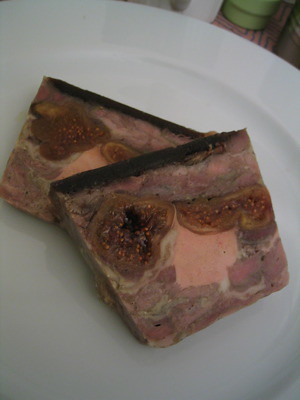On a round, white ceramic plate set upon a flat surface, there are two thick, square-shaped slices of what appears to be a meat pie or similar dish. The pieces are stacked, with one leaning against the other. The top of each slice is a darker brown, possibly indicating a crust or slight charring. The insides reveal varied colors and textures: shades of brown, light pink, and some white, reminiscent of marbled meat, as well as gooey, yellowish-brown chunks, possibly cheese. Additionally, there are visible pieces that could be specialty olives and various other ingredients. No bites have been taken from the slices. The overall colors on the plate range from dark browns and light browns to pink and yellow, with hints of white. Towards the upper right of the plate, a green item—potentially a cup—can be seen. No people are present in the image.